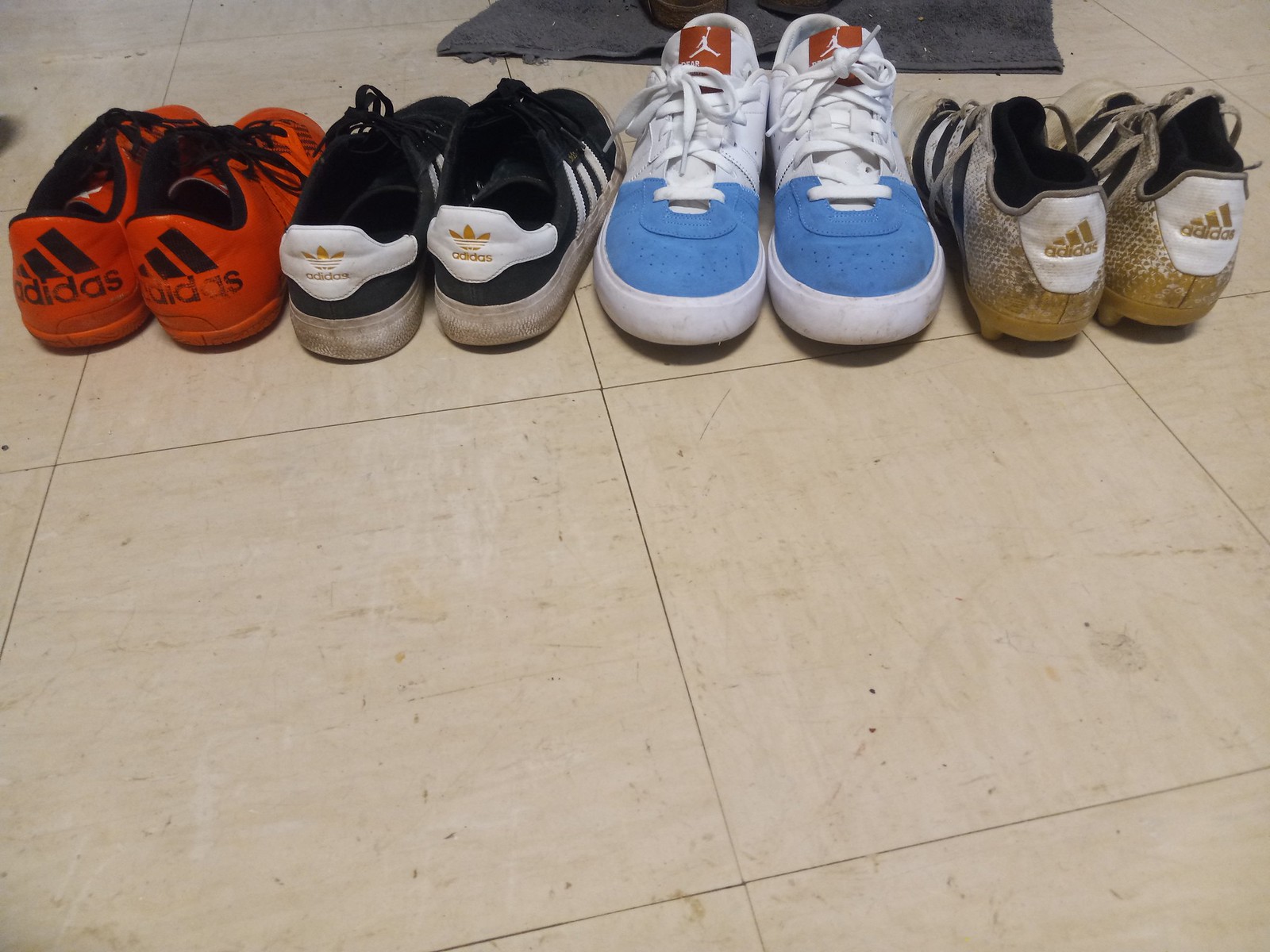In this color photograph, we see a dirty, tiled floor featuring large, square tiles in a marbled white and tan color, with black spots and dust. On the top half of the image, four pairs of well-worn sneakers are neatly lined up. Moving from left to right, the first pair are bright orange Adidas sneakers with black interiors and laces, prominently displaying large black Adidas logos on their backs. The second pair are dark blue (or possibly black) Adidas shoes featuring three white stripes on the sides and a white heel with a gold Adidas logo. These shoes have a dirty white base. The third pair are white and blue Jordans, with a blue toe box and tongue, white midsections, and brown Jordan logos on the tongues. The final pair are predominantly white Adidas sneakers with gold spots on the backs and gold Adidas logos, embellished with three black stripes on the sides. Just behind the lined-up shoes, a partially visible dark gray towel sits, with the bottoms of a pair of black shoes peeking out from underneath, hinting at more footwear beyond the picture’s frame.